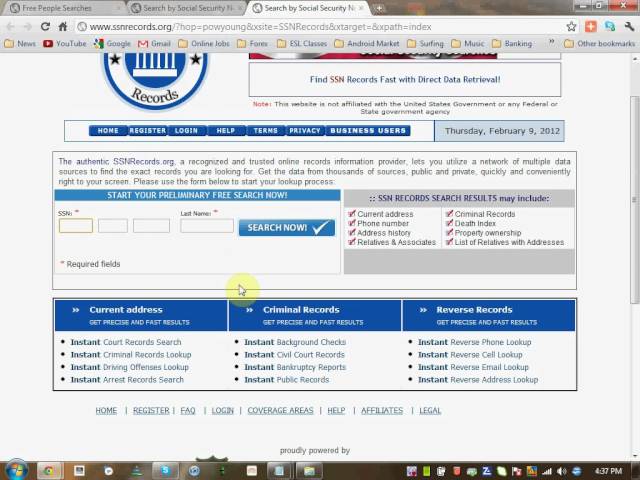A detailed screenshot showcases a desktop screen running on the Windows Vista operating system, identifiable by the signature glassy "Start" button featuring a marble-like Windows logo in the bottom left-hand corner. The primary focus of the screenshot is a web browser, tentatively identified as Google Chrome, displaying the website SSNrecords.org.

The webpage itself displays a white background adorned with an official logo near the top, partially obscured due to the screen being slightly scrolled down. Prominent text reads, "Find SSN records fast and with direct data retrieval," positioned towards the right side of the page. Below this, a navigation bar consists of several blue rectangular tabs with white text, labeled: Home, Register, Log In, Help, Terms, Privacy, and Business Users.

Beneath the navigation bar, a search box invites users to input a Social Security Number and last name. This facilitates the retrieval of comprehensive information records, potentially including an individual's address, phone number, address history, relatives and associates, criminal records, death index, property ownership, and a list of relatives with their respective addresses.